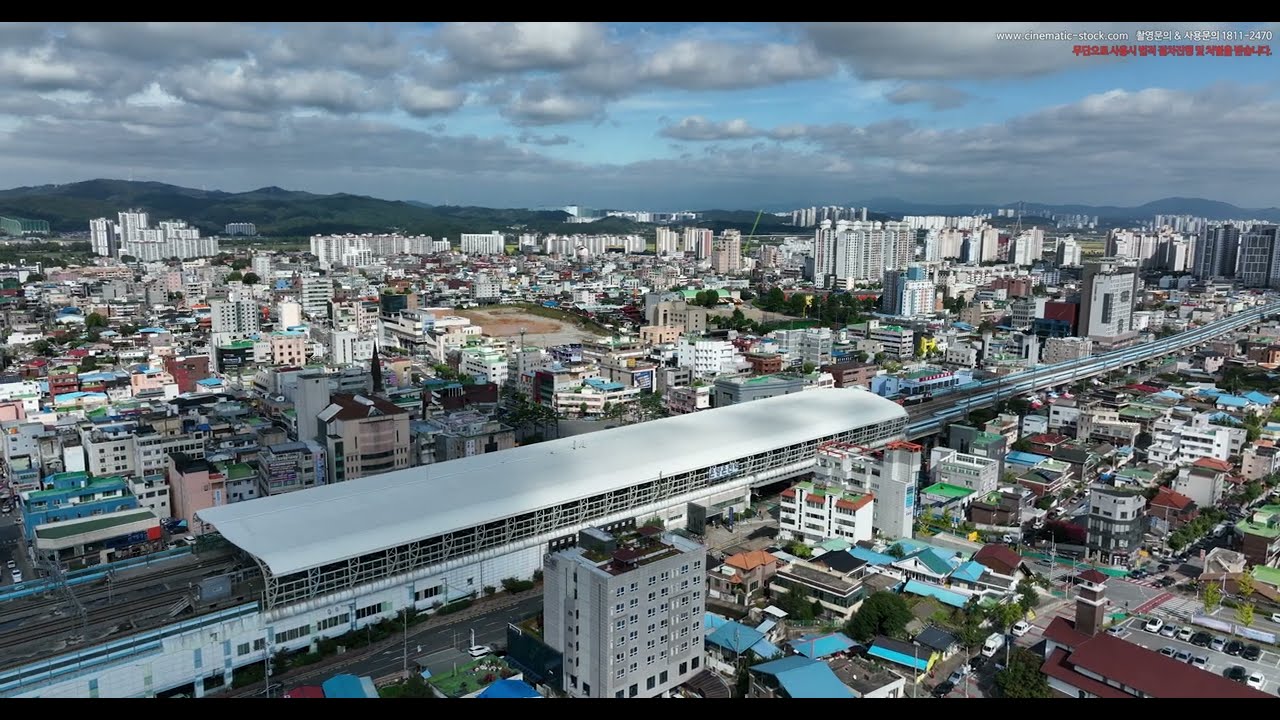This aerial, full-color photograph captures a large and densely populated city under an overcast sky. The image prominently features a network of city buildings, ranging from mid-sized structures to taller buildings about 20 stories high, though none are true skyscrapers. A significant portion of the cityscape includes blue-roofed smaller homes and apartment buildings, possibly indicative of a shantytown or tent city. 

Running diagonally from the bottom left to the upper right is a busy freeway, partially covered by a large white roof supported by metal caging, suggestive of a light rail pickup and drop-off area. Streets and parking lots filled with vehicles are evident throughout the bustling city scene. In the background, rolling hills and silhouetted mountains form the horizon, adding a natural contrast to the urban landscape.